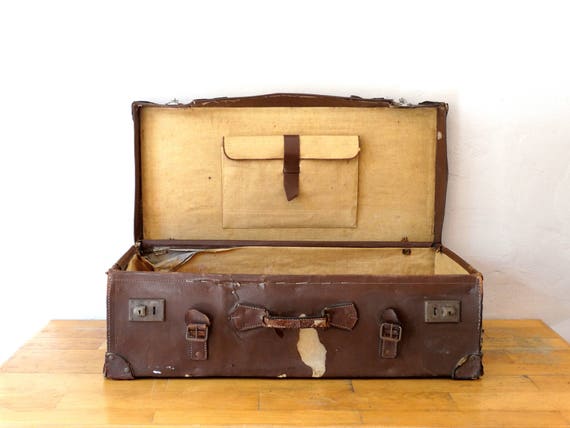The image features a horizontally aligned, rectangular, old-looking suitcase set against a white, slightly textured wall. The suitcase, which appears to be made of dark brown leather and is visibly worn, sits atop a light wooden table with a brick-like pattern. The suitcase is open, revealing its contents. At the front, a brown handle is present, positioned above a large rip that exposes a light brown or cream-colored material underneath. On each side of the suitcase, there are two silver latches and buckles. The inside of the lid has a worn appearance and features a file-folder-style pocket. The light source seems to come from overhead, casting shadows towards the right, accentuating the aged and deteriorating state of the leather on the top edge and the left side of the suitcase.